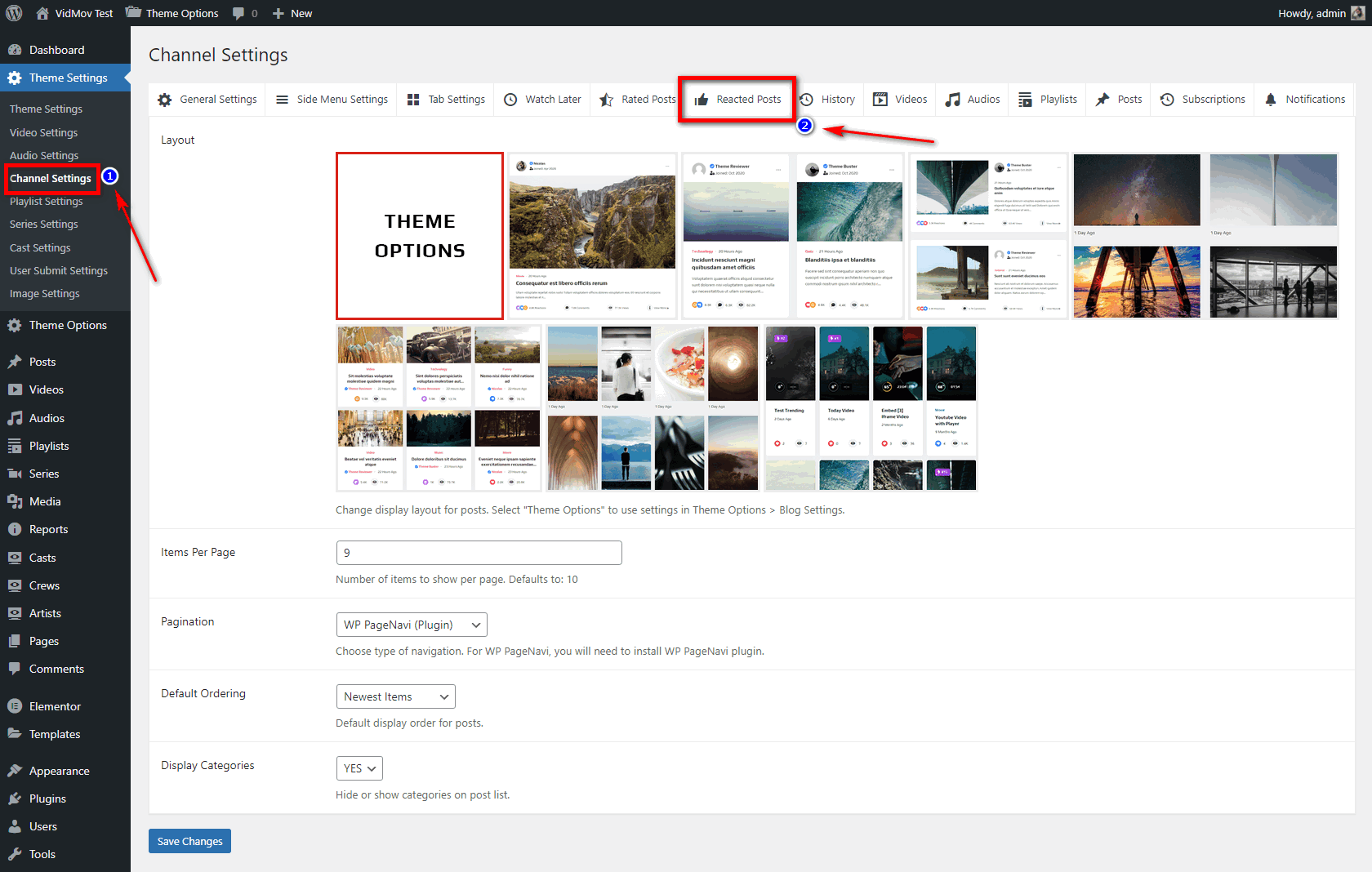The image depicts a webpage interface resembling a dashboard for managing content or settings. The upper left-hand corner features multiple logos, including one labelled "VidMore," followed by an unreadable word, and a house icon. Adjacent to these elements are a speech bubble icon, another logo, a plus symbol, and the word "New." On the right-hand side, the page is identified by the username "Rowdy Admin" with an associated logo.

The left-hand section of the interface is dominated by a thick black vertical band, functioning as an index or navigation bar. This side includes various icons and labels, starting with "Dashboard" represented by a speedometer icon, followed by "Theme Settings" denoted by a gear icon. Below "Theme Settings" is the "Channel Settings" option, which stands out with a gray background. 

On the main, white page area bordered in gray, there's a blue button situated at the bottom left corner. Within this page, multiple setting options are listed, beginning with "General Settings." There appear to be approximately 12 options available. Additionally, the interface seems to include multiple pages displaying different images. A notable feature is a red box highlighting certain posts, possibly redacted, accompanied by an arrow.